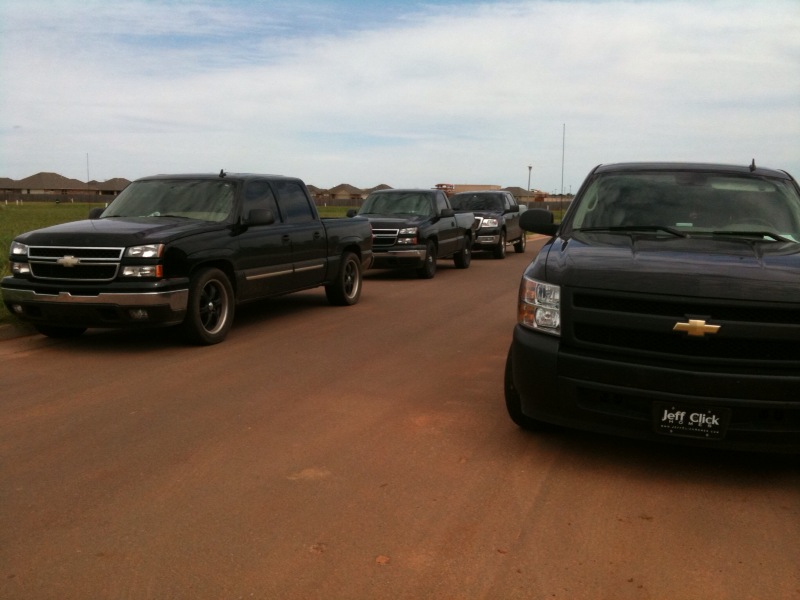The image captures a long line of predominantly black pickup trucks parked along a smooth, wide orange dirt road, taken from a slight angle that makes the road appear wider in the foreground. On the left side of the road, three black pickup trucks are clearly parked, while on the right side, the front end of another black pickup truck, prominently displaying a front plate that reads "Jeff Click," partially obstructs the view of any vehicles behind it. The background features a lush green grassy field, extending to a distant row of small brownish mountains. The sky above is light blue, scattered with thin, plentiful white clouds.